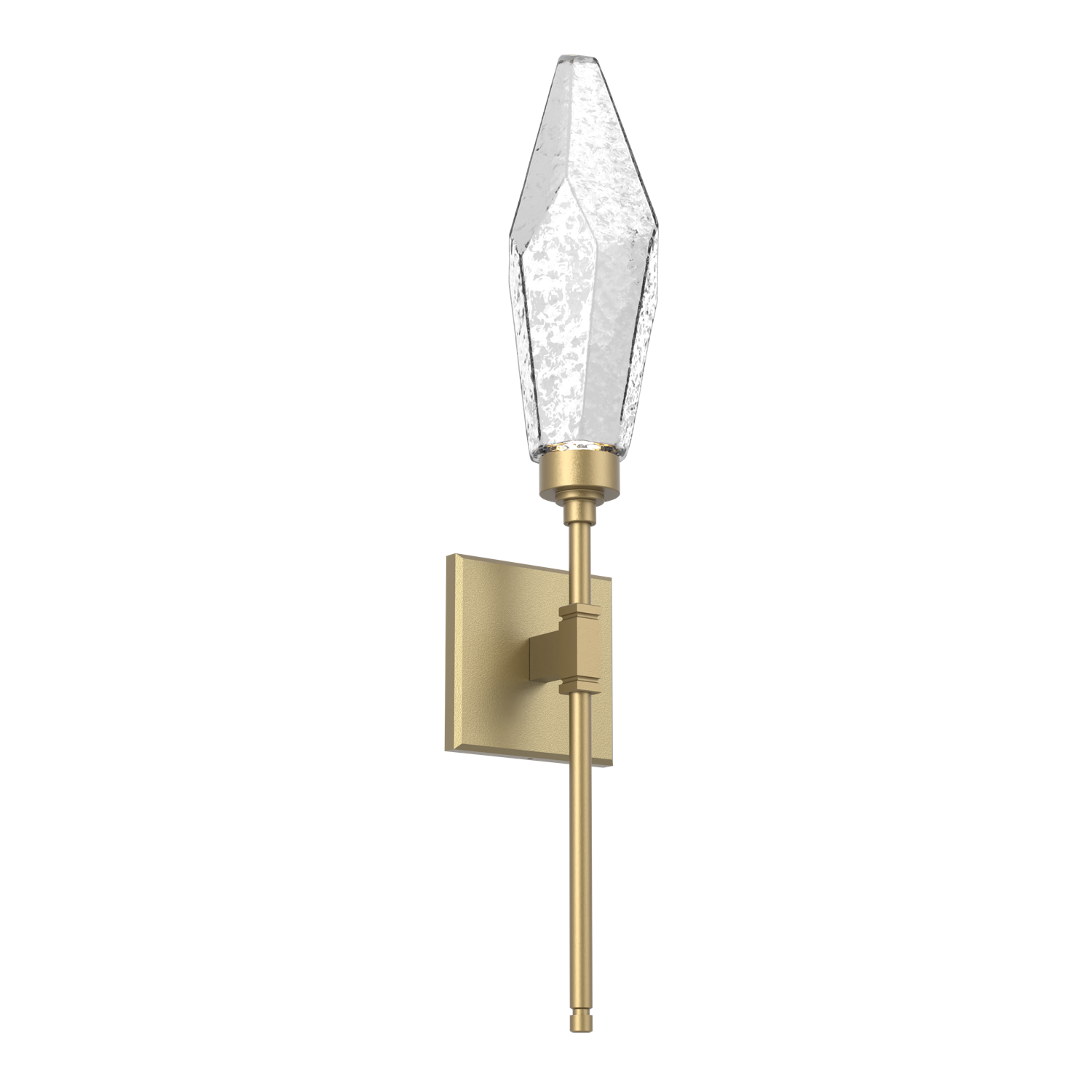The image depicts a unique wall-mounted lamp with an intricate design. The lamp is affixed to the wall via a square, gold-colored bracket, which gives it a regal and sturdy look. The main body of the lamp has a cylindrical shape, reminiscent of a royal scepter, further enhanced by the gold elements that connect it to the wall. The lamp itself has a frosted crystal top, shaped like a pointed spear, adding to its torch-like appearance. The design suggests a blend of elegance and functionality, making it both a decorative piece and a practical fixture. The background is nonexistent, implying that this is likely a stock image of the product for retail purposes.